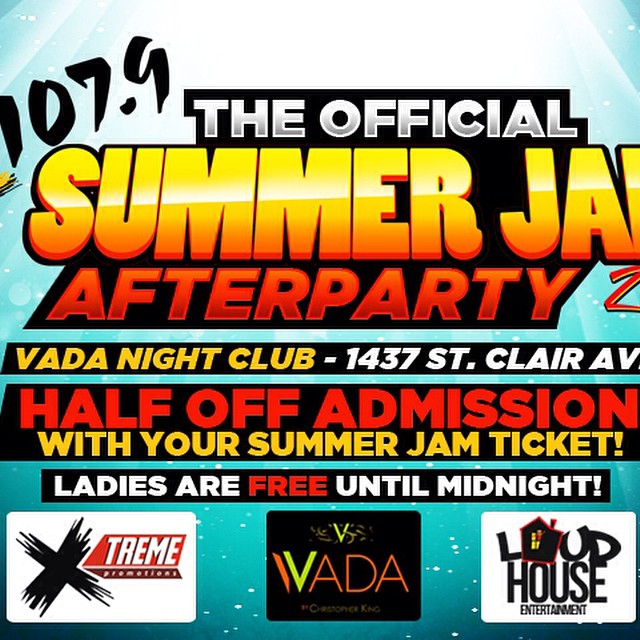This image is a close-up of a square promotional flyer with a turquoise-to-white gradient background, which gives the impression of a light shining down from the top. The text at the top of the flyer prominently reads "107.9" followed by "The Official Summer Jam After Party 2." This main title features a dynamic color scheme: "The Official" is in white, "Summer Jam" has a yellow-to-orange gradient, and "After Party" is in red. Below this heading, three black bars contain further details. The first bar reads "Veda Nightclub, 1437 St. Clair Ave" in white text. The second bar states "Half-off admission with your Summer Jam ticket," where "Half-off admission" is in red and "with your Summer Jam ticket" is in yellow. The last bar announces "Ladies are free until midnight," using white text with "free" highlighted in red. Towards the bottom, the flyer features three rounded logos: "Xtreme Promotions," "Veda" accompanied by the name "Christopher King," and "Loud House Entertainment," the latter of which incorporates a house image in the 'O' of "Loud." The edges of the flyer are slightly cropped off, cutting off some details. The various colored texts and the gradient background give the flyer a vivid, summery vibe, perfect for the event's theme.